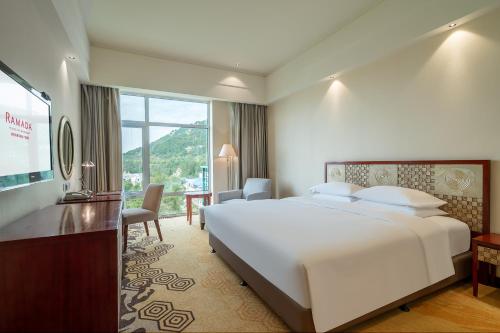The image depicts a well-appointed hotel room at the Ramada, captured in a rectangular frame that is wider than it is tall. The room is dominated by a king-sized bed with an elegant oversized headboard and four meticulously arranged pillows, all dressed in crisp white linens. Illuminating the space are stylish sconces mounted on a protruding section of the wall above the bed. The tan carpet with intricate brown designs adds warmth to the room's predominantly white color palette. 

On the left side of the room, there is a substantial brown dresser topped with a wall-mounted TV displaying the Ramada logo in red. Next to the dresser, a wall mirror and a desk with a chair provide practical and aesthetic appeal. Completing the furnishings is a recliner situated in the right-hand corner of the room, offering a spot for relaxation. The far wall features an expansive, floor-to-ceiling window with gray curtains opened to reveal a picturesque view of green hillsides, trees, and grassy areas. This detailed depiction showcases the room's harmonious blend of comfort, style, and scenic beauty.